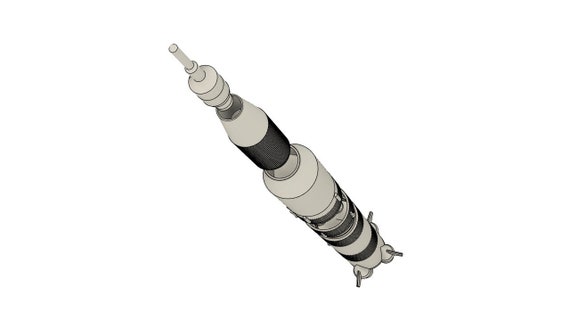This digitally created, black and white rendering features a complex rocket-like device viewed from a top angle, descending from the lower right to the upper left corner of the image. The rocket is composed of approximately six distinct sections, beginning with a narrow, pointed tip, followed by a neck that transitions into a composite cylindrical body. The body itself consists of layered components: two donut-shaped rings, a white and black striped cylinder, a wider cylinder adorned with alternating black and white bars, and finally, a base supported by three legs, suggesting it could stand independently. The grayscale color scheme includes varying shades from light gray to almost black, contributing to the intricate detailing of this sophisticated, unidentified tool or device.